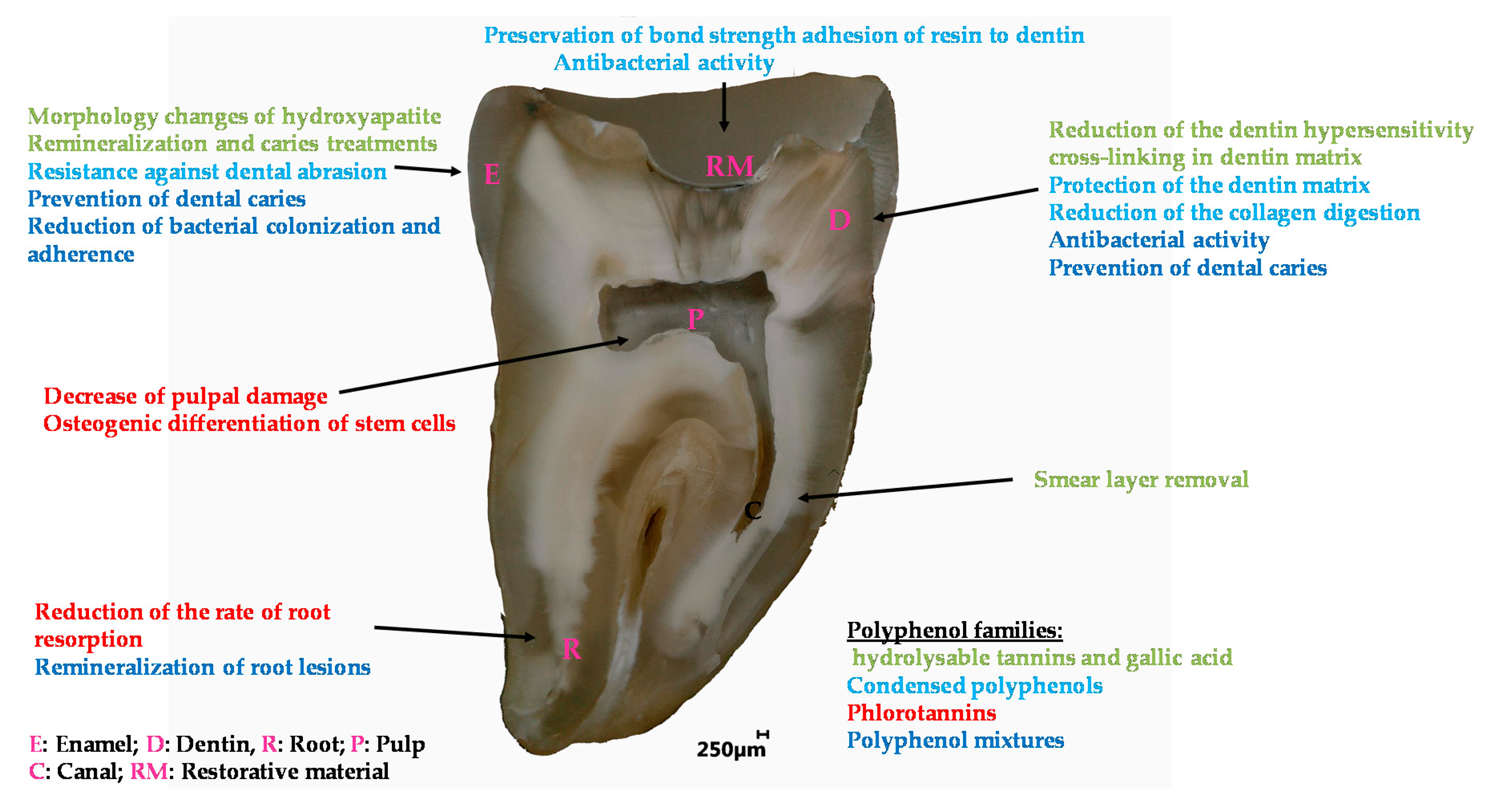This detailed illustration of a tooth, suited for a dental textbook or classroom poster, features a bisected tooth, revealing its internal structure for educational purposes. The cutaway view, rendered in dark brown, highlights various layers such as the enamel, dentin, root, pulp, and canal, along with restorative materials. Different colors—greens, blues, and reds—are used to delineate and describe distinct parts and processes. 

The top of the image emphasizes "Preservation of Bond Strength" and "Adhesion of Resin to Dentin," integrating discussions on antibacterial activity. Detailed labels specify parts of the tooth like enamel and root, each accompanied by informative descriptions that explore processes like hydroxyapatite morphology changes, remineralization, and treatments for cavities. The diagram also details the reduction of dentin hypersensitivity and smear layer removal, emphasizing the tooth's preservation and restoration. 

Overall, the illustration serves as a comprehensive guide to understanding tooth anatomy and dental restoration techniques, making it an essential educational tool for dental students and instructors.